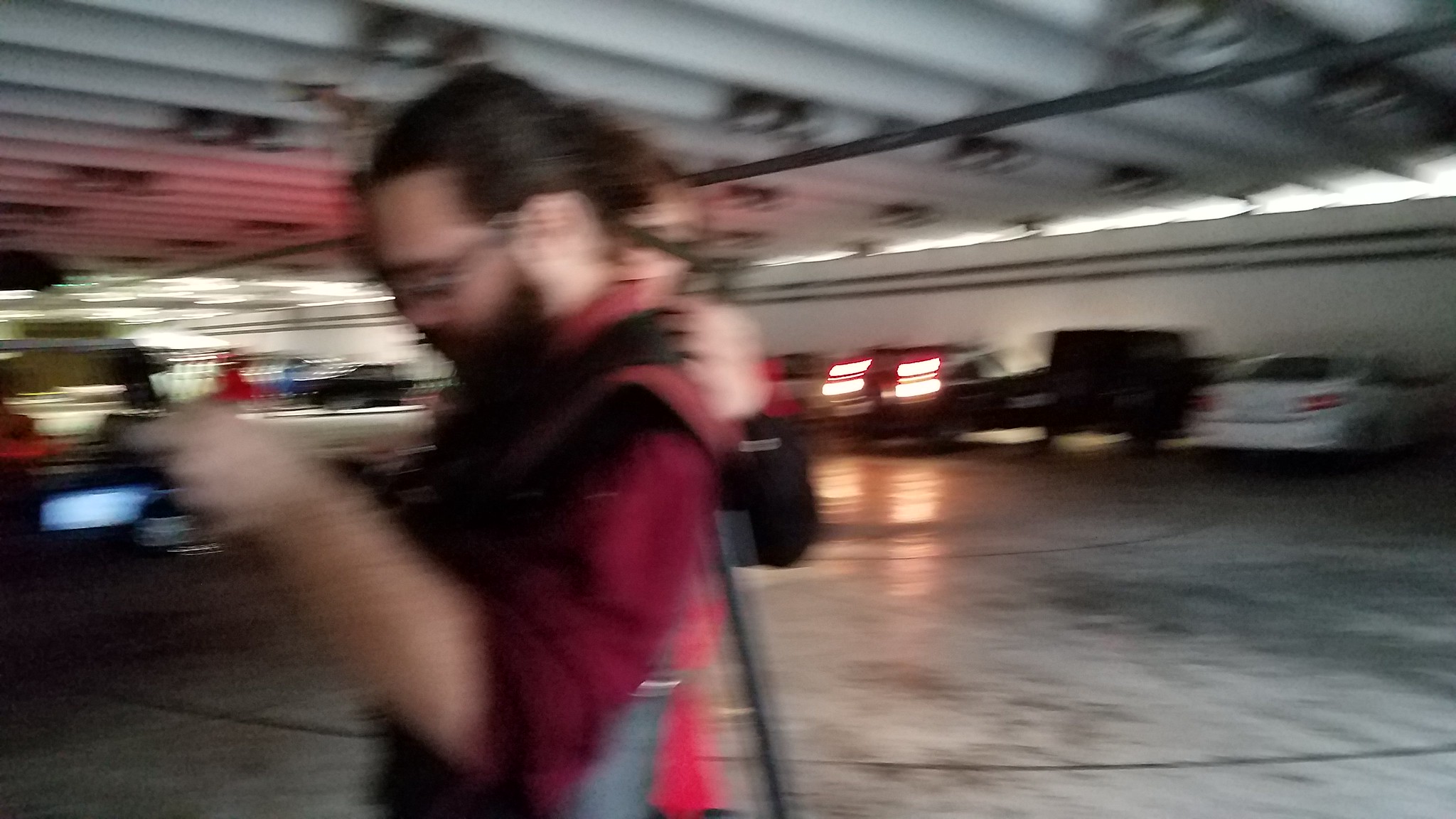In this photograph taken in a parking garage, the central figure is a Caucasian man with a beard and glasses, who is looking down at his phone. His hair is tied back in a ponytail, and he is dressed in a red shirt with black or gray accents. A partially visible hand rests on his back, suggesting the presence of another person who appears to be wearing a black jacket but remains out of view. The background is an indoor parking garage, illuminated by both natural sunlight and fluorescent lights. Various cars occupy the space, including one that seems to be reversing, as indicated by its illuminated lights. The cars are of different colors, including white, black, and possibly a dark shade of blue. The overall scene is dominated by gray and black tones of the parking structure. The image is quite blurry, making specific details difficult to discern.